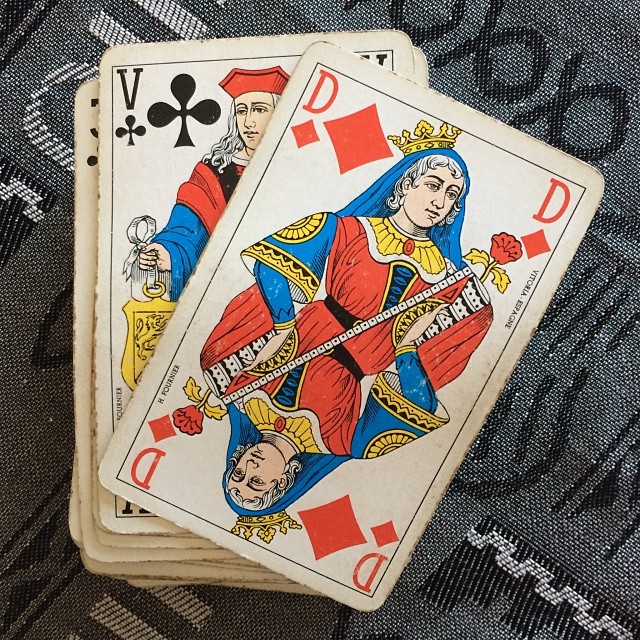In the image, the first noticeable feature is the background, which appears to resemble either a textured rug or a thick placemat. The background is primarily dark gray, interspersed with hints of white, elongated black lines, shorter black lines, and white rectangular patterns. 

In the lower left corner of the image, there are additional white rectangles adorned with thin gray lines. Shifting our focus to the center, we see a playing card featuring a figure who appears to be a king from a different era. This figure is adorned with a crown and a blue scarf on their head, has shoulder-length gray hair that curls outward, and is dressed in an ornate top comprising red, gold, and blue elements. Prominently displayed on this card is the red letter "D," flanked by red diamond symbols on either side.

Below this card and slightly to the left, there is another card marked with the letter "V" and a club symbol, both in black. This card depicts a different character, wearing a red colonial-style hat and possessing long, curly gray hair. This character is holding a gold emblem featuring a lion.